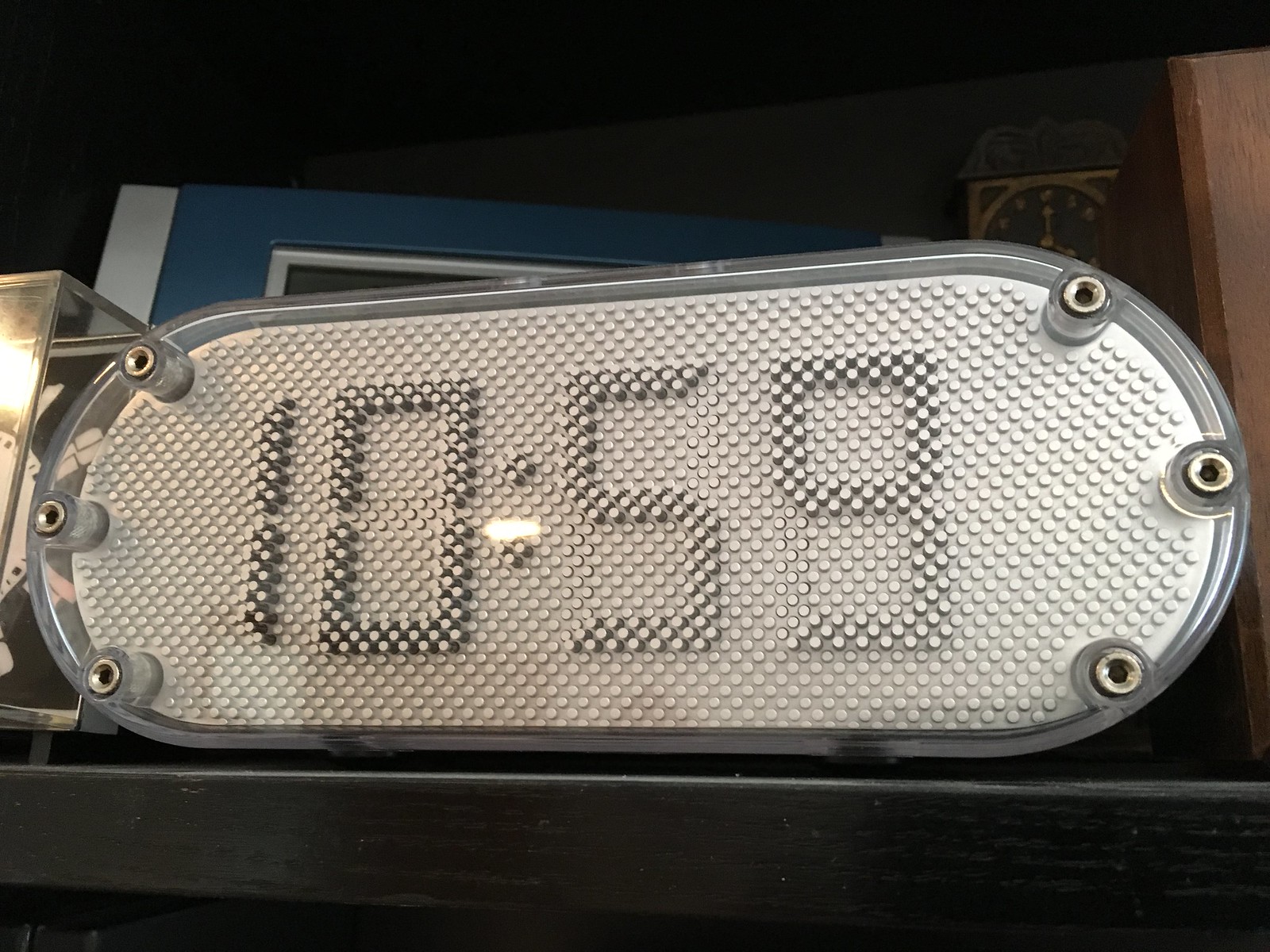In this close-up photo, a digital oblong clock is prominently displayed on a black wooden shelf or table. The clock features a clear plastic casing with a silver face that has a distinctive textured surface made up of numerous tiny dots. The time displayed on the clock reads 10:59, with each number composed of small round pegs, adding to the clock's intricate design. Behind the clock, another item with a blue plastic body and a white door or border is partially visible, adding a splash of color and context to the scene.